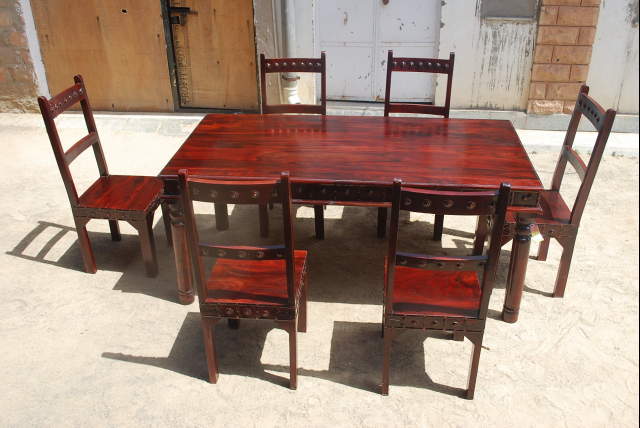The image captures a striking outdoor setting featuring an ornate cherry-red wooden dining table accompanied by six matching chairs. The table, richly carved around the edges, and the chairs are arranged with two on either side and one at each end. The scene appears to be in front of a building with exposed red brick and a white concrete ground underfoot, casting distinct shadows due to the bright daylight. Behind the dining set, there is a rustic wooden gate with a black iron latch and a painted white warehouse door, further enriched by an artistic splatter of paint. This eclectic backdrop suggests the location might be at the rear of a warehouse or an auction house. The combination of the grand furniture and the industrial background creates a unique and intriguing composition.